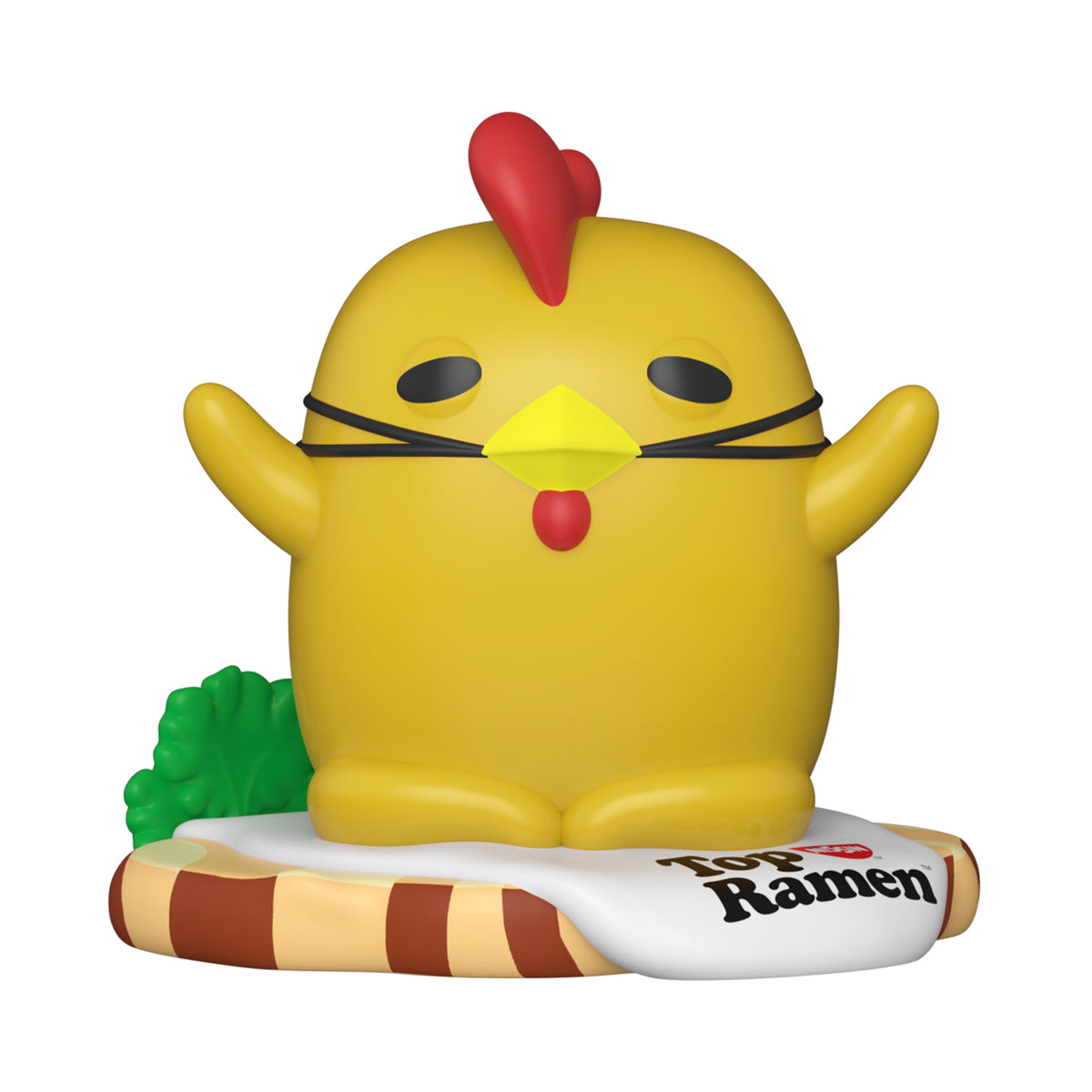The image presents a detailed photograph of what appears to be a plastic figurine of the Top Ramen mascot, resembling a comical, egg-shaped chicken. The vibrant yellow mascot features a prominent red mohawk and a peculiar red goatee beneath its beak. Its beak is tied up with strings, enhancing its playful, almost mask-like appearance. The chicken has expressive black eyes and uplifting arms, emitting a joyous demeanor. Positioned on a white background, the mascot stands atop a brown base that has darker brown striping, reminiscent of a hamburger patty. Surrounding the base, green leaves suggest a touch of garnish, enhancing the overall visual appeal. Below the mascot, the Top Ramen logo is prominently displayed, stamped on what looks like an egg yolk. The entire setup hints at either an AI-generated image or a collector's item and maintains a childlike, charming aesthetic, perfect for display.